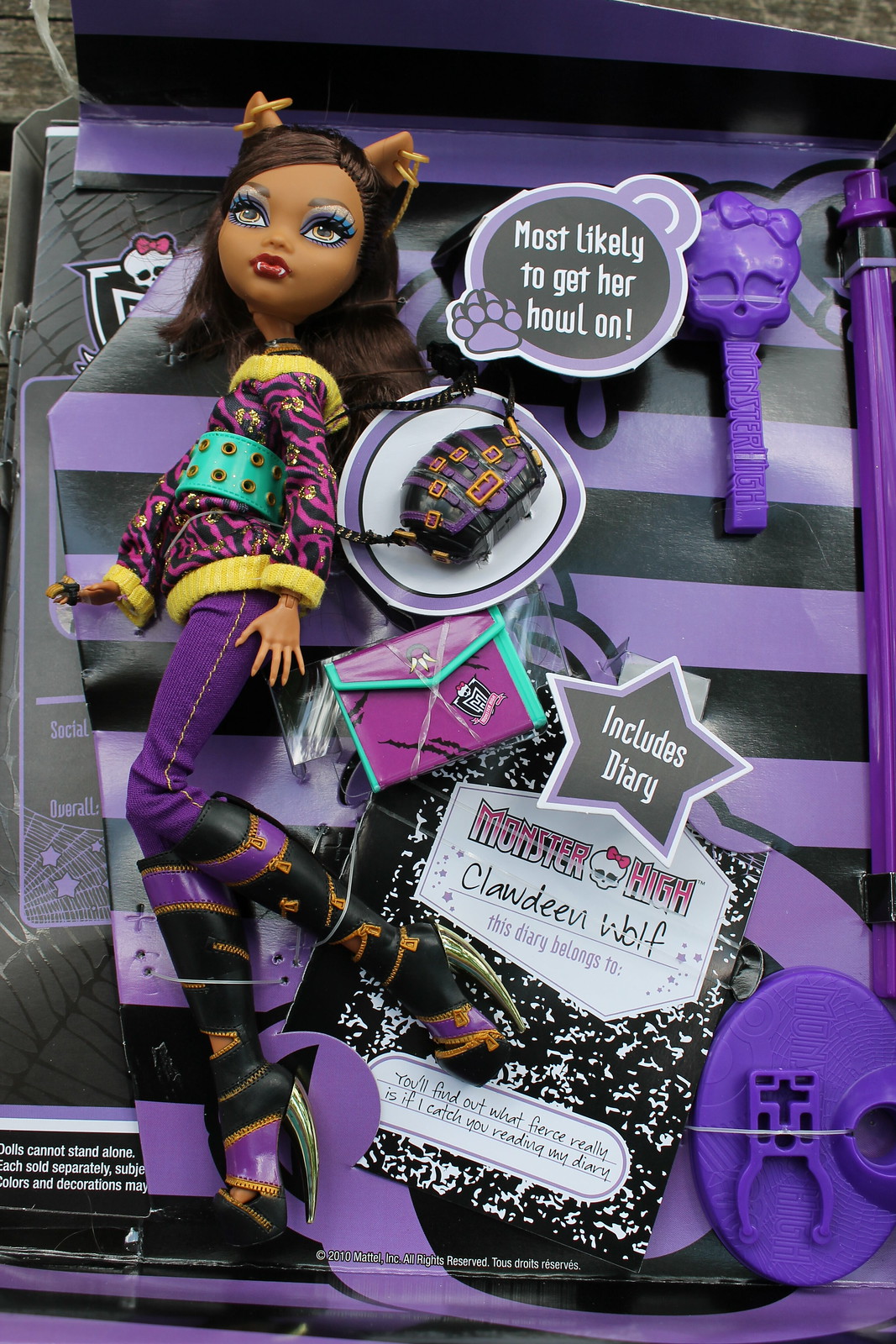The photograph depicts a child's toy doll still encased in its packaging. The vibrant packaging is designed with dark purple and black stripes, contributing to a spooky yet playful gothic theme. This doll is part of the Monster High franchise and is prominently labeled "Claudine Wolf." The brand name "Monster High" is featured near the top of the box in bold text along with the tagline, "most likely to get her howl on," suggesting a werewolf-inspired character.

The doll, with a dark complexion and striking makeup, including blue and light purple eye accents and visible fangs, has a distinct look. She sports dark brown, shoulder-length hair, and wears an animal print pink and black jacket, purple pants, and matching purple and black boots adorned with gold accents. A bright green belt adds a pop of color to her outfit.

The packaging includes several accessories neatly arranged around the doll. Among them are a small purse, a paper bag, a hair tie featuring a skull, and a notebook inscribed with "Monster High, Claudine Wolf" and the phrase "includes diary." A pencil or pen, likely purple, is also visible, enhancing the playset's completeness. The overall presentation is clearly aimed at young children who are enthusiasts of Halloween-themed or spooky characters.